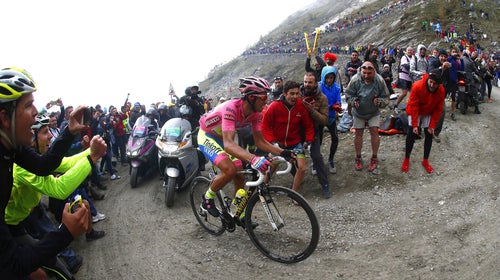This captivating color photograph captures the excitement of a bike race ascending a rocky, gravel-strewn hill. The sky in the top left remains a blank canvas, enhancing the focus on the vibrant scene below. Dominating the foreground, a determined cyclist in a striking red helmet and jersey, complemented by neon yellow pants with blue and pink accents, pedals uphill through an energetic crowd. His white-handled bike contrasts sharply against the earth-toned path. The trail is swarmed with spectators donning colorful attire—red and green coats stand out amongst the sea of supporters, all cheering fervently. Trailing closely behind the lone cyclist are two motorcycles, possibly police or race escorts, adding to the intensity of the moment. The hillside is packed with enthusiastic fans, a testament to the event's excitement and the cyclist's valiant effort.